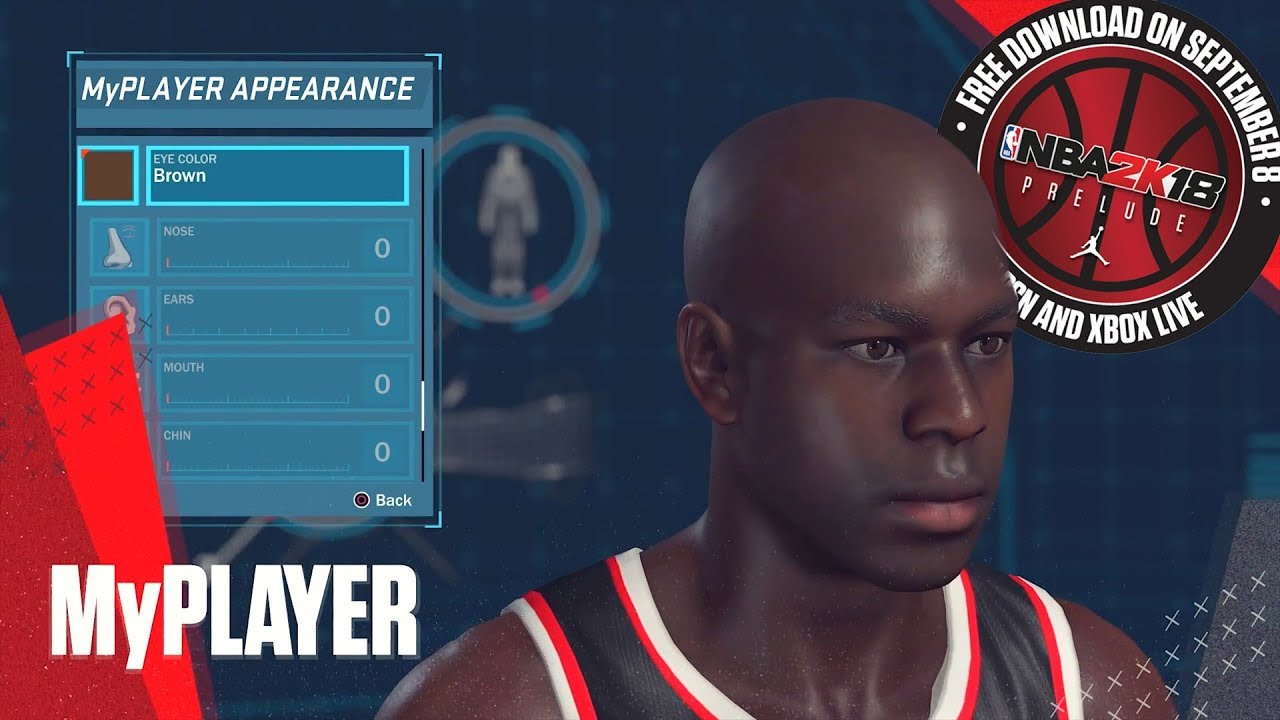The image appears to be a promotional screenshot from the video game NBA 2K18, specifically detailing player customization options. On the left side, within a long blue box, the text "My Player Appearance" is prominently displayed at the top. Beneath this header, a blue square outlines a brown color with the label "Eye Color: Brown" to the right. Below this section, icons for a nose and an ear are labeled "Nose" and "Ear," respectively, demonstrating further customization features.

In the lower left corner, another section marked "My Player" in bold white text against a red background is visible. Adjacent to this, an avatar of a basketball player is shown, featuring brown skin, brown eyes, and clad in a sleeveless jersey with white, red, and black colors, though only the upper portion is visible.

The upper right corner highlights the text, "Free Download on September 8th, Xbox Live," indicating a special downloadable content release date. Central to the image is a black and red basketball with the text "NBA 2K18" written in the middle, followed by "Prelude" underneath. The iconic NBA logo, featuring a white silhouette of a basketball player leaping with a ball, is also displayed, reinforcing the game's branding.